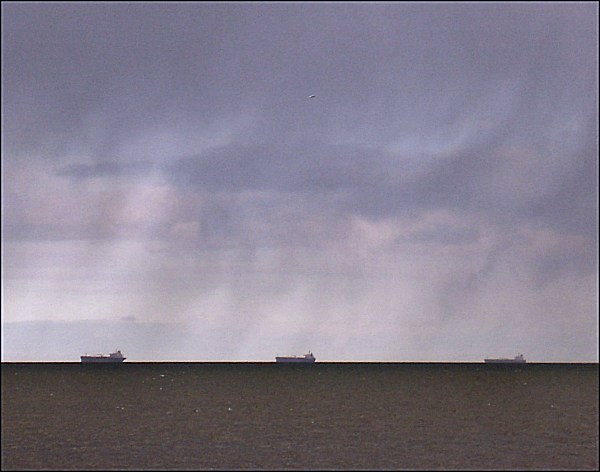This captivating photograph showcases a tranquil seascape under a dramatic sky. The upper two-thirds of the image is dominated by a purplish, cloud-filled sky, accented with patches of white and streaks of gray descending towards the ocean, suggesting impending heavy rain. Below, the ocean itself is a solid dark gray, with subtle ripples indicating light movement but overall appearing calm and undisturbed. 

On the horizon, where the sea meets the sky, three large ships are clearly visible, equally spaced from left to right. Their white or possibly grayish-blue forms suggest they are likely empty cargo vessels, oil tankers, or naval ships, given their substantial size and shape. The photo’s atmospheric tones make it difficult to discern whether it's a color image subdued by weather conditions or captured in monochrome.